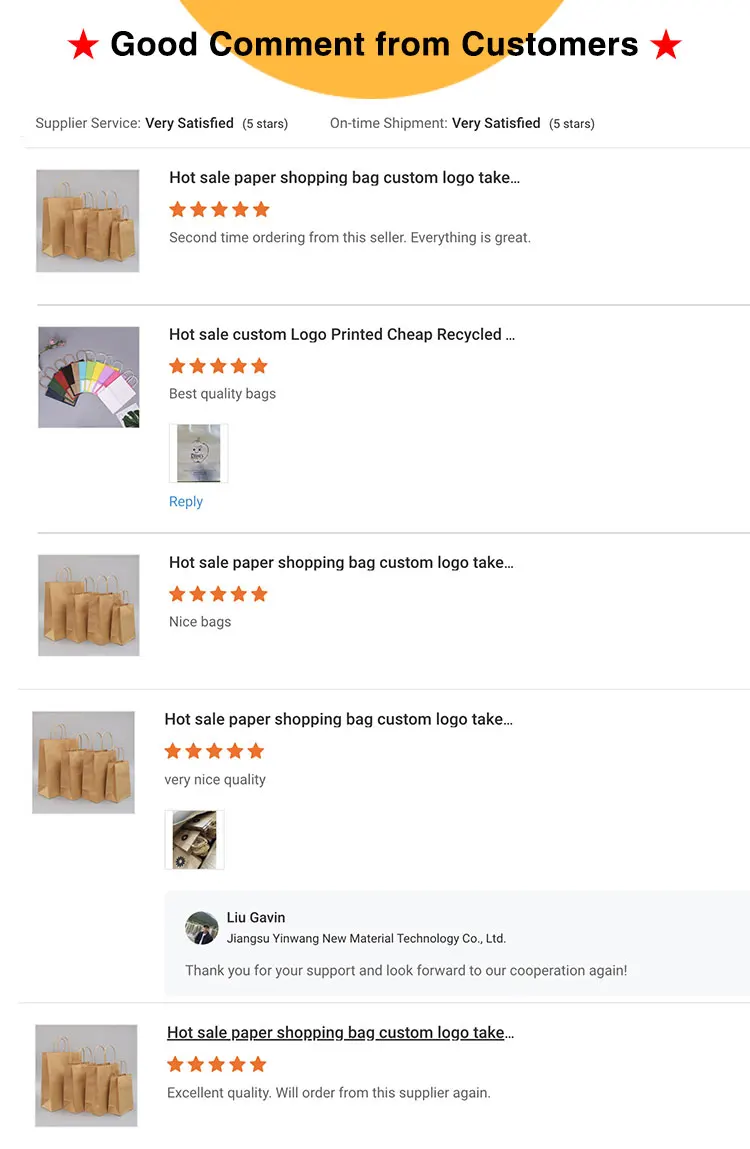This image, sourced from a review website, showcases a detailed layout of user feedback. The top two inches of the image feature a blank white space, followed by a thin gray border. Approximately an inch and a half below, there's a section containing a user review, framed by another gray border of about two inches. This pattern continues, with each review section having its own gray border. In total, there are four separate reviews presented.

At the top of the image, a segment of a yellow circle, resembling the lower quarter of the Sun, is visible. Overlaying this circle, there's a prominent red star next to bold black text that reads, "Good Comment From Customers." Below this text, in smaller letters, the words "Supplier Service" are displayed.

Running down the left side of the image are several small pictures. The first image depicts five grocery bags, followed by an image of key chains. The next three images are similar, all displaying grocery bags. Adjacent to these images, in bold black text, are various comments such as "Very Satisfied Five Stars" and "On Time Shipment Very Satisfied Five Stars," spaced out evenly.

To the right of each image, there is additional information. For example, the first image has a blue square background with brown bags, next to which black text reads, "Hot Sell Paper Shopping Bag Custom Logo..." Below this, five yellow stars indicate a positive rating, and under that in smaller text, it states, "Second time ordering from the seller. Everything is great." This format is repeated for each review, with each having a gold star rating and a comment. The fourth review also features a response indicated by a small blue bar, showing a reply from a company representative with the name "LIUGAVIN."

This image effectively captures the essence of user feedback, complete with visual aids and detailed commentary.